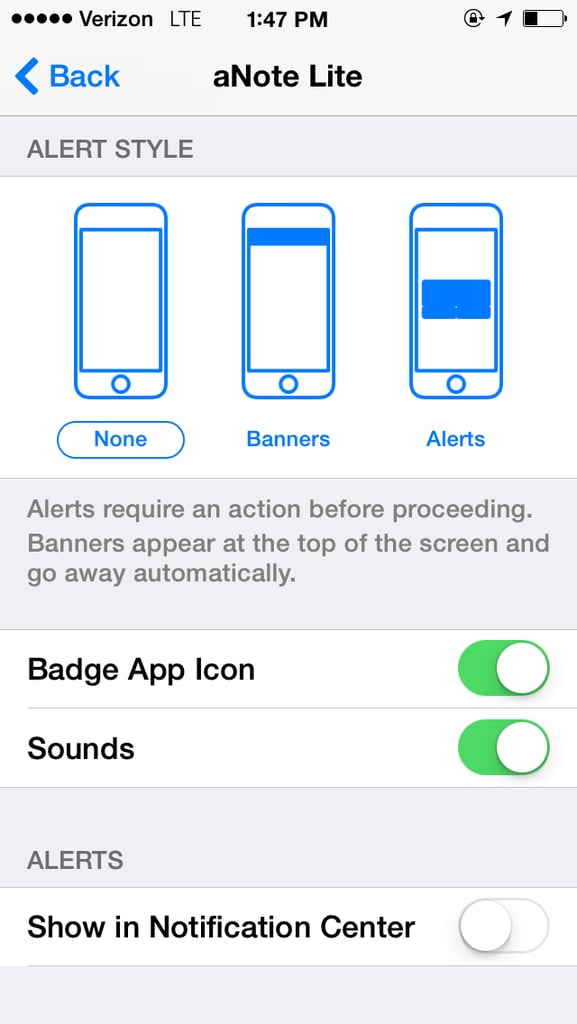Screenshot from a smartphone displaying the AnoteLite app interface. At the top of the screen, the status bar shows five signal circles, Verizon LTE network, 1:47 PM, screen lock icon, a share or navigation icon, and a battery level at roughly 30%. 

Below the status bar, a navigation bar includes a blue “Back” button accompanied by blue text that says “Back,” and the title “AnoteLite.” The main content of the screen shows an "Alert Style" selection with three outlined iPhone silhouettes representing different notification styles. 

The first silhouette on the left, labeled "None," is highlighted with a capsule shape. The middle silhouette is labeled "Banners," showing a dark blue line at the top of the screen. The third silhouette is labeled "Alerts," with blue floating panels depicted in the middle of the screen. 

A description in gray text beneath the options clarifies: "Alerts require an action before proceeding. Banners appear at the top of the screen and go away automatically." 

Below this, there are two toggle buttons: the first one for "Badge App Icon," which is turned on, and the second for "Sounds," also turned on. Further down, another section titled “Alerts” includes a toggle for “Show in Notification Center,” which is currently turned off. Each section is divided by thin, one-pixel gray lines.